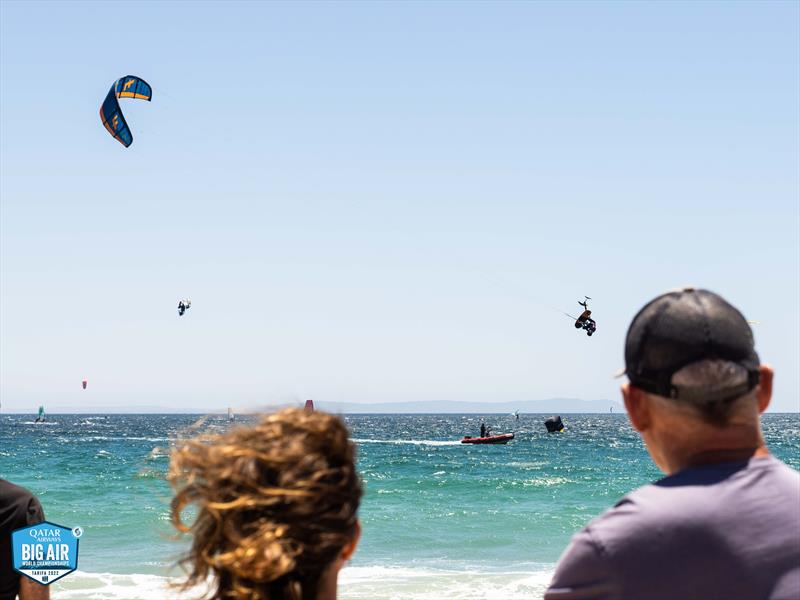A vibrant, horizontally-oriented photograph captures a sunny day at the beach, showcasing an engaging beach sport event. In the foreground, we see the backs of two spectators: a woman with blonde hair on the left and a man wearing a black hat and a purple shirt on the right, both gazing intently at the activity in the ocean. A distinctive blue diamond-shaped logo in the lower left corner reads "Qatar Big Air" in bold white letters, indicating the event's name.

The sparkling greenish-blue ocean on the bottom third of the image is adorned with white waves gently washing up on the pristine, crystal white sand. The water is alive with action, featuring four kite surfers skillfully maneuvering in the air, some appearing to perform flips. A boat cutting across the scene from left to right leaves a prominent wake behind it, helmed by a man who seems to be assisting the airborne skiers. The boat's presence adds dynamism to the event as it supports the kite surfers' acrobatics. 

Above the water, dominating the top two-thirds of the photo, is a clear, stunning blue sky with no clouds, enhancing the overall energetic and fun atmosphere of the beach event. In the distant horizon, a faint silhouette of a landmass is just visible, completing the picturesque coastal scene.